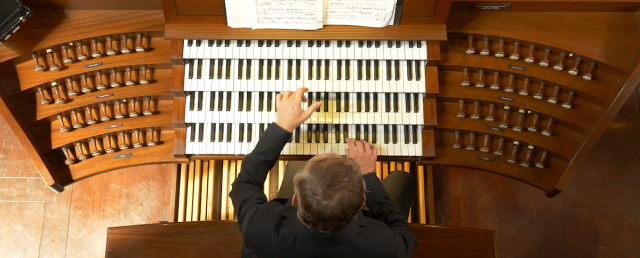An overhead view captures a middle-aged man with light brown hair and a black long-sleeved shirt, sitting on a wooden bench and playing an elaborate organ. The organ features four offset keyboards, each fitted with black and white keys. The man’s right hand is poised on the lowest keyboard, while his left hand reaches between the second and third rows. Above the keyboards, an open music book with black writing is positioned, though the text is too small to decipher. The organ and surrounding area are predominantly wooden, including the floor, which transitions from an orange-tinted section with a white light shining on it to a very dark brown area. Wooden structures resembling cabinets with wooden shafts and silver balls are present on either side of the organ. In the upper left corner of the image, a black plastic box with a silver opener is visible. The scene is detailed and richly textured, emphasizing the wooden aesthetic throughout.